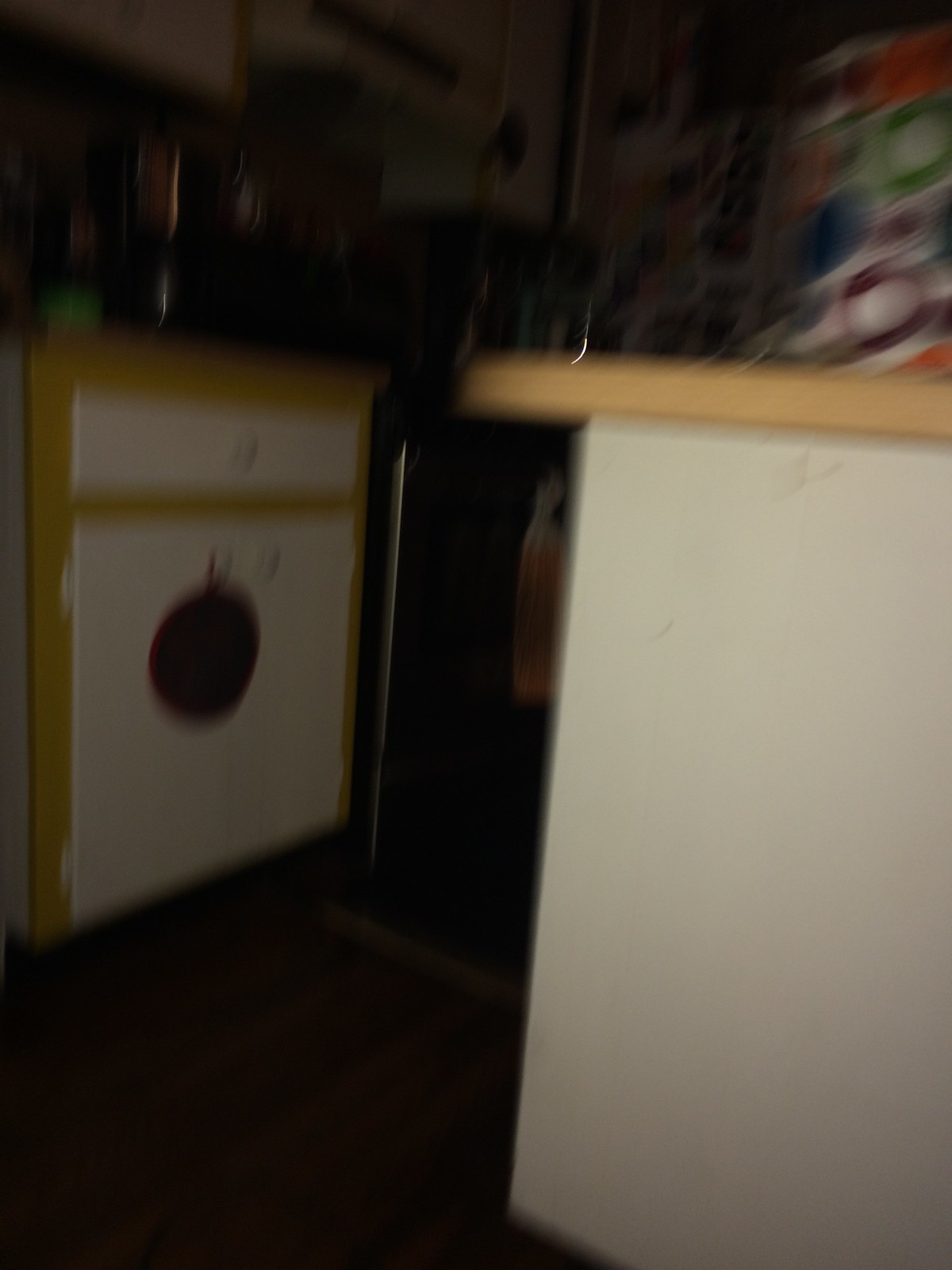The blurry image depicts an interior space, likely a kitchen or break room. Central to the image is a small appliance resembling either a mini dishwasher or a clothes washer, characterized by its yellow sides, trim, and a white door with a white drawer on top. Opposite this machine is a counter with a white side panel and a light brown, particle board top. On this counter, there's a shopping bag decorated with rainbow-colored circles. Adjacent to the small appliance is a brown stove, accompanied by a range hood and some white cupboards above. There is also a coffee pot situated above the stove and the appliance. The lighting is dim, making it challenging to discern finer details.